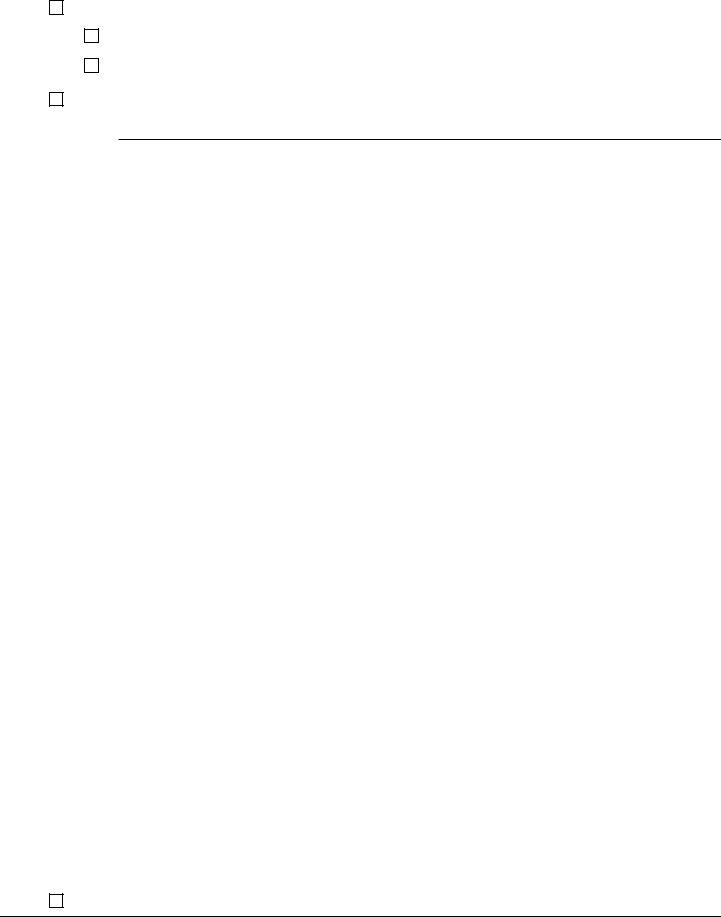In the screenshot, there are two distinct lawns. The top lawn is slightly shorter in length. To the left of this lawn, there are four sequentially positioned squares that form a semi-circular pattern. The first square is located at the far left edge. Moving down to the second row, the second square is positioned slightly farther out to the right. The third square, found in the third row, is further out still, maintaining alignment with the previous squares but progressing outward. The fourth square in the pattern is significantly lower, aligning beneath the first square at the top.

Below the top lawn, there is a second lawn. On the left side of this bottom lawn, there is another square that is in alignment with both the first and fourth squares of the top lawn, creating a coherent visual symmetry between the two lawns.